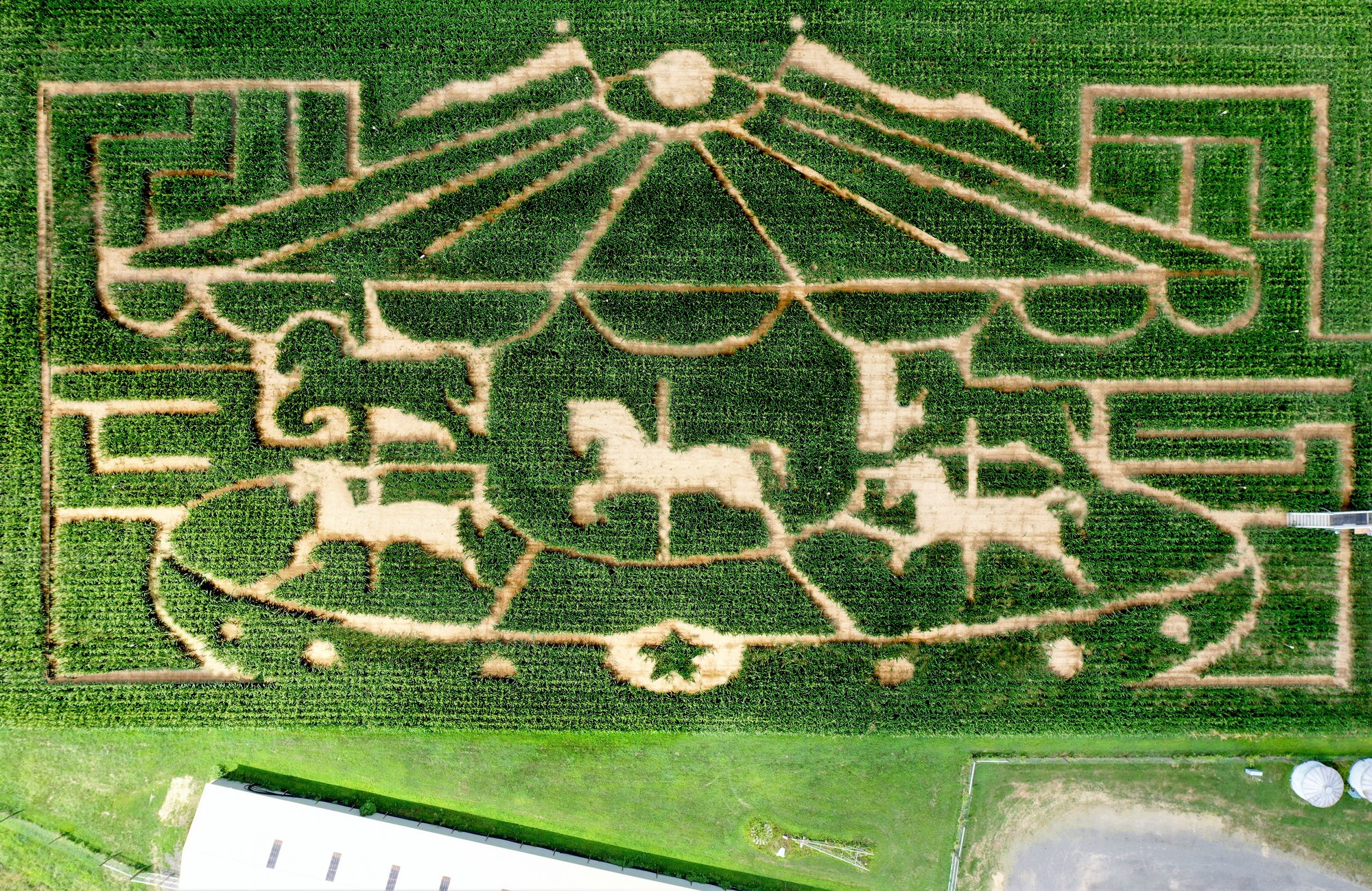The image depicts an aerial view of a large field where the crops have been meticulously cut to create an intricate design resembling a carousel. The depiction includes a rounded carousel top adorned with long flags, a circular base, and finely detailed horses on poles positioned in the center and at corners of the carousel. The design is prominently outlined, giving the carousel a striking appearance against the green expanse of the crops, with the carousel itself being white in color. A star is carved at the bottom, adding to the complexity and beauty of the artwork. The background also features parts of a farm building and possible water tanks, indicating the rural setting. Despite the realistic and detailed appearance, it’s challenging to determine if this is an actual photograph or a highly detailed artistic rendering.